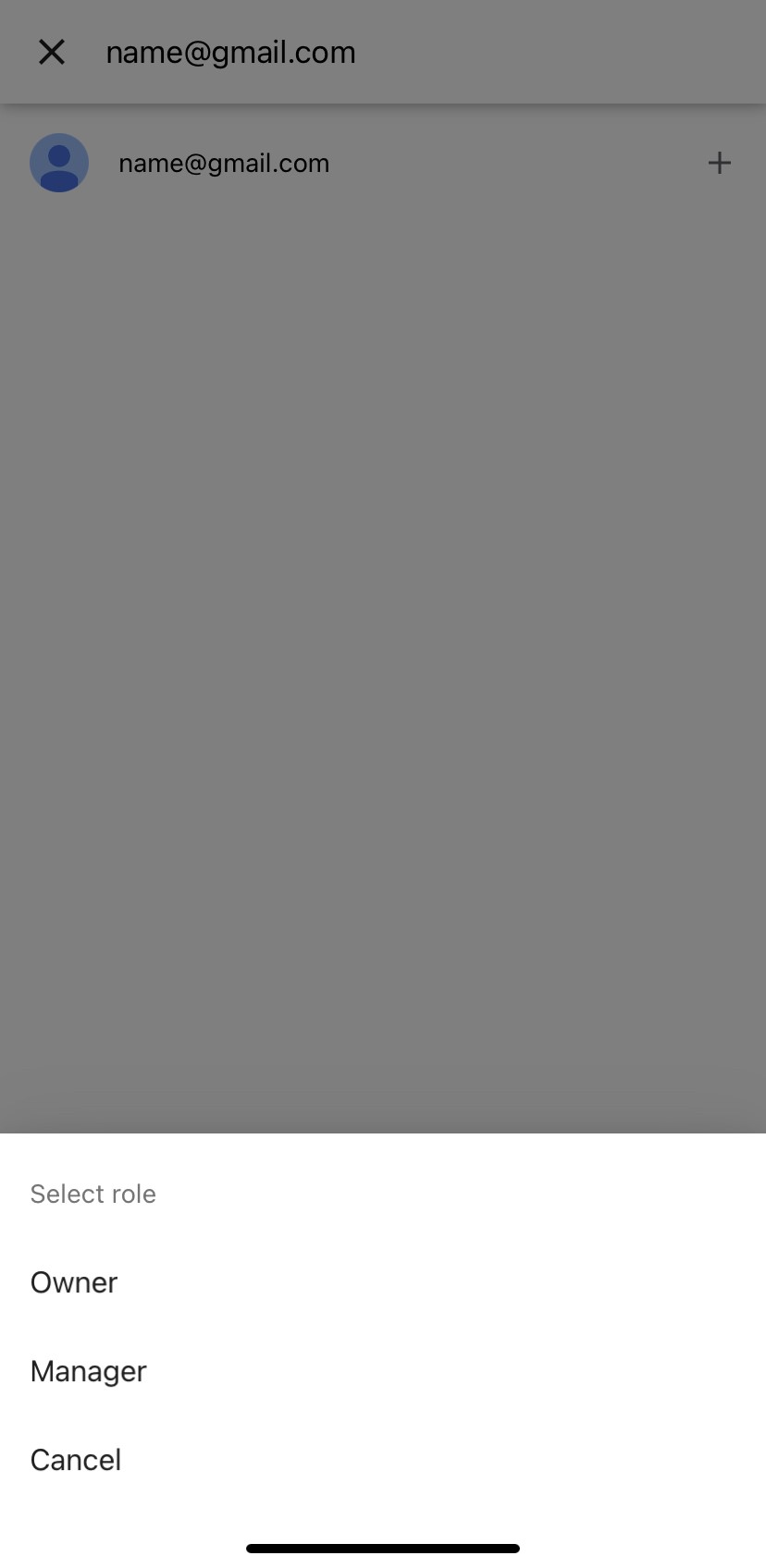In this screenshot taken from a mobile device, the background features a predominantly white canvas with the top two-thirds of the image exhibiting a grayish overlay. At the very top, a bar stretches across the screen, starting with a black "X" in the left-hand corner, which serves as a close button. To its right, in all lowercase black print, the text "name@gmail.com" is displayed.

Directly below this bar, on the left-hand side, is a circular blue icon featuring a darker blue silhouette of a person, indicating a blank profile picture. Adjacent to this icon, the same email address, "name@gmail.com," is repeated in black lowercase text. On the far right-hand side of this section, a small plus sign encourages users to add a new contact.

Below this segment is a vast expanse of blank space, creating a visual divide. In the lower third of the image, which lacks the gray overlay, a pop-up window with a white background appears. The heading in gray print reads "Select Role." Beneath this heading, three role options are listed in black text: "Owner," "Manager," and "Cancel." Finally, a black line cuts horizontally through the middle of this bottom section, providing a clear demarcation within the image.